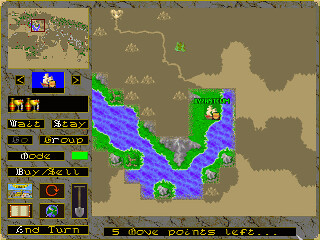This image is a pixelated screenshot from an old-style video game, resembling classic SimCity graphics. The main portion on the right showcases a map, with a vibrant, explored section in the middle forming a reverse J shape. This area displays bright green grass and a medium blue river, contrasting with the dark brown and light tan unexplored lands. The upper left panel features a mini-map of the larger game world, highlighting in red the specific segment currently visible on the main map. Below this panel, there's a dark blue rectangular landscape with an indiscernible image in the center. Adjacent are long rectangular buttons labeled “Wait,” “Stay,” “Group,” “Mode,” and “Buy/Sell.” The lower left corner contains various icons, including a shovel, a red circle, and a book-like symbol, alongside another button for “End Turn." At the bottom of the map section, a black rectangle displays the text "Five more points left…", all in beige-colored text. The retro, slightly blurry aesthetic suggests an early-generation game, possibly showing a gameplay screen with interface elements for player commands and game stats.